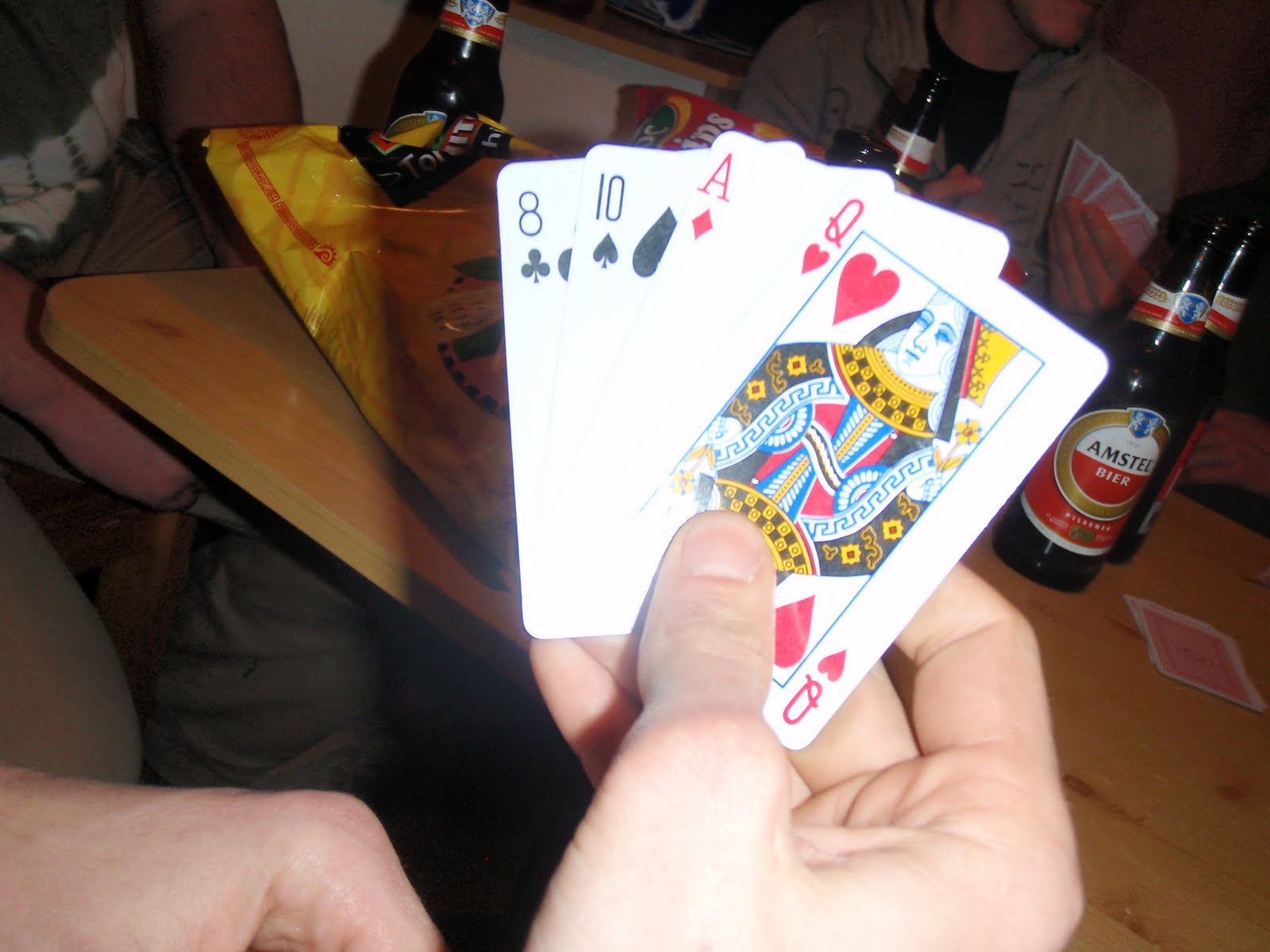A hand is prominently featured in the center of the image, holding up four playing cards. The cards are fanned out in a semi-circle configuration beneath the person's thumb and rest atop the fingers, which are tucked underneath. The topmost card is the Queen of Hearts, followed by the Ace of Diamonds, which is partially obscured. Next is the Ten of Spades, and finally, the Eight of Clubs. A portion of the person's hand is visible in the bottom left corner, showcasing their knuckles and part of their index finger pointed downward.

In the background on the right side, there is an amber-colored beer bottle with a label that includes a gold circle enclosing white and red sections, bearing the name "Am Steel Beer." The cards and bottle rest on a light yellow wooden table scattered with more playing cards, visible only from the backs.

In the distant upper right corner of the image, another person is seen with their head turned to the right, revealing only their chin. This person is dressed in a gray shirt over a black undershirt and is also holding four cards. A beer bottle is positioned directly in front of them.

To the left, behind the main set of cards, a yellow bag with red stripes at its base is partially visible, adding a splash of color to the scene.